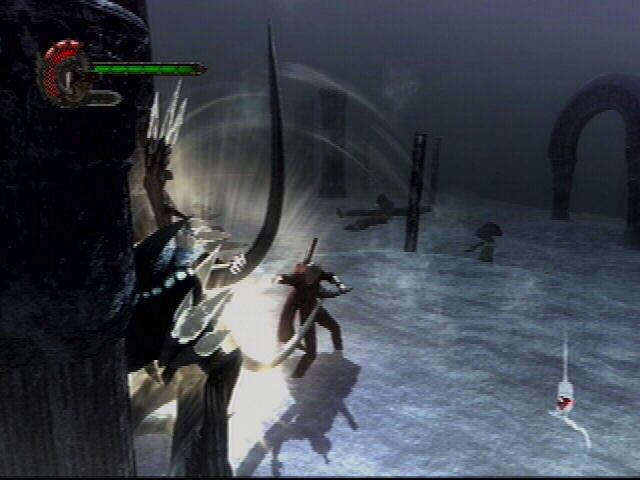This is a detailed screenshot from a fantasy-themed video game, reminiscent of titles from the early 2000s. In the upper left corner, there is a sword icon adorned with lines and a green hue, likely representing life force or health. Adjacent to the sword icon is a C-shaped dragon icon featuring red and brown colors, possibly indicating a secondary status or power meter. At the bottom of the screen, several fighters are depicted, each adorned with sharp, antler-like protrusions. The ground beneath them is shrouded in a foggy, white ambiance, while the sky above is a dark, ominous gray, nearly black. In the background, arches punctuate the horizon, adding to the game's mystical and ancient atmosphere.